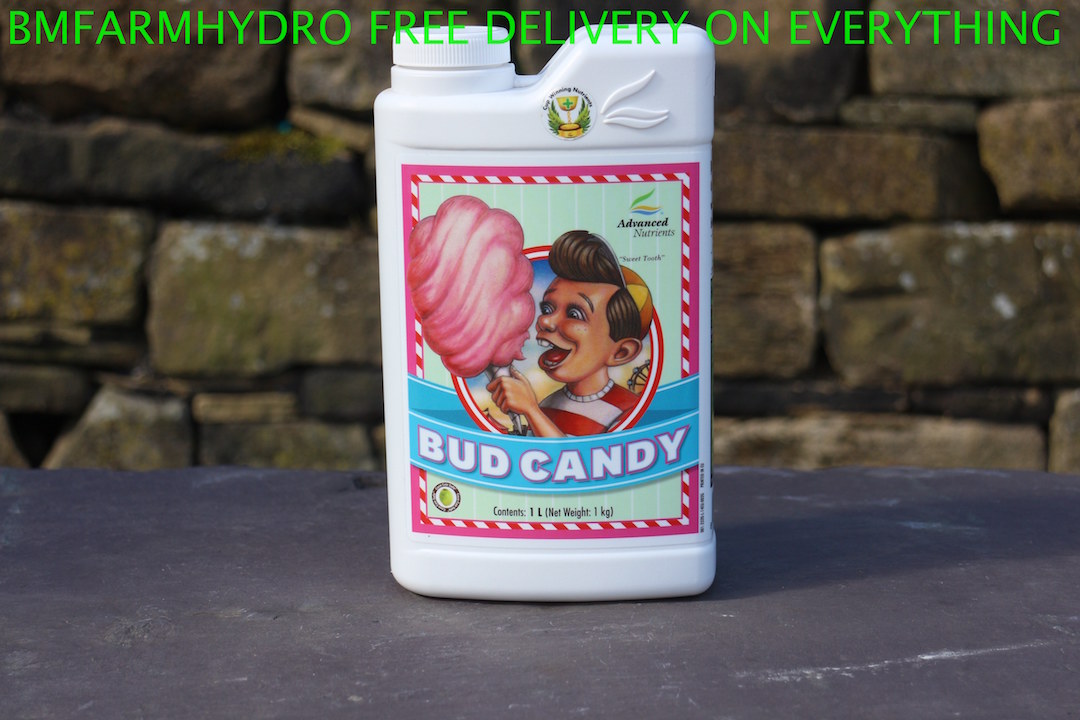This detailed image features a white bottle labeled "Bud Candy" prominently displayed on a table with a brick building in the background. The bottle's label is adorned with a vibrant illustration of a young boy wearing an orange and yellow cap along with a red and white striped shirt, holding a pink cotton candy and appearing eager to take a bite. The boy has freckles on his cheeks, adding to the playful and nostalgic imagery. Above the illustration, the bottle boasts "Cup Winning Nutrients" and "Advanced Nutrients Sweet Tooth," and at the bottom, it specifies "Contents One Liter, Net Weight One Kilogram." The label itself has a pink border, followed by red and white candy stripes, set against a green background with white stripes, further enhancing its eye-catching appearance. Additionally, text on the bottle includes "Bee Farm Hydro, Free Delivery on Everything." The entire scene captures a blend of whimsy and practicality, reminiscent of childlike delight juxtaposed with essential gardening supplies.